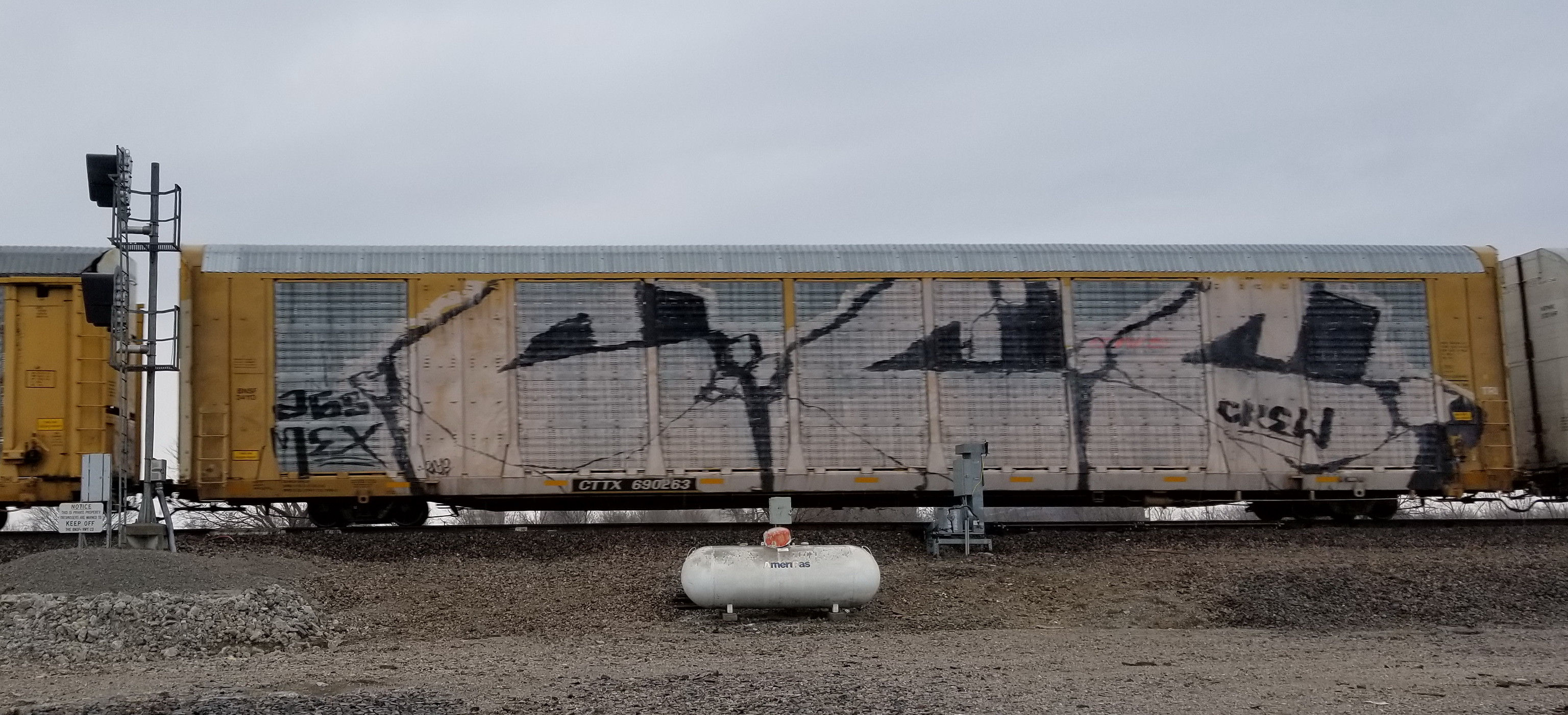The image depicts a section of train tracks on a gray, overcast day. The ground is barren, featuring dirt, rocks, and bits of coal, devoid of any grass or plants. Positioned several feet away from the tracks is a white or whitish-gray tank embedded in the ground with some dirt on top. The tank resembles a propane tank. The focal point is a series of three train cars, with one prominently centered and the other two partially off-frame. The central and right-most train cars are a yellowish, golden color with silver on top, while the car to the center-right appears to be white or off-white. All three cars are covered in assorted graffiti, including bold, black, and white letters and symbols. Notably, the graffiti on the center car could spell out something like "CCC crew" or "444 crew," with various other tags scattered alongside. A "Notice: Keep Off" sign is also visible next to the tracks, enhancing the sense of an industrial, abandoned setting.